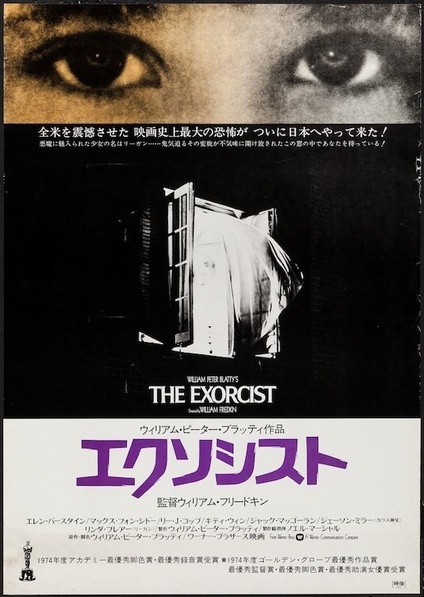This is a detailed poster for the movie "The Exorcist," primarily featuring text in what appears to be Japanese. Dominating the top quarter of the poster is a striking pair of eyes: the left eye is portrayed in a yellowish tone, while the right eye and the nose are highlighted in stark black and white. Below these haunting eyes, the middle section of the poster presents an eerie black background showcasing an open window with white light streaming through, accompanied by billowing curtains. Centered beneath this imagery, in both English and Japanese text, is "William Peter Blatty's The Exorcist," with "The Exorcist" prominently displayed in purple katakana script. This section is framed by additional Japanese text providing more context about the movie. In the bottom left-hand corner of the poster, an Academy Award statue is visible, suggesting the film's critical acclaim. Most of the descriptors and titles on the poster are rendered in Japanese script, adding an Asian cultural twist to this iconic horror film advertisement.